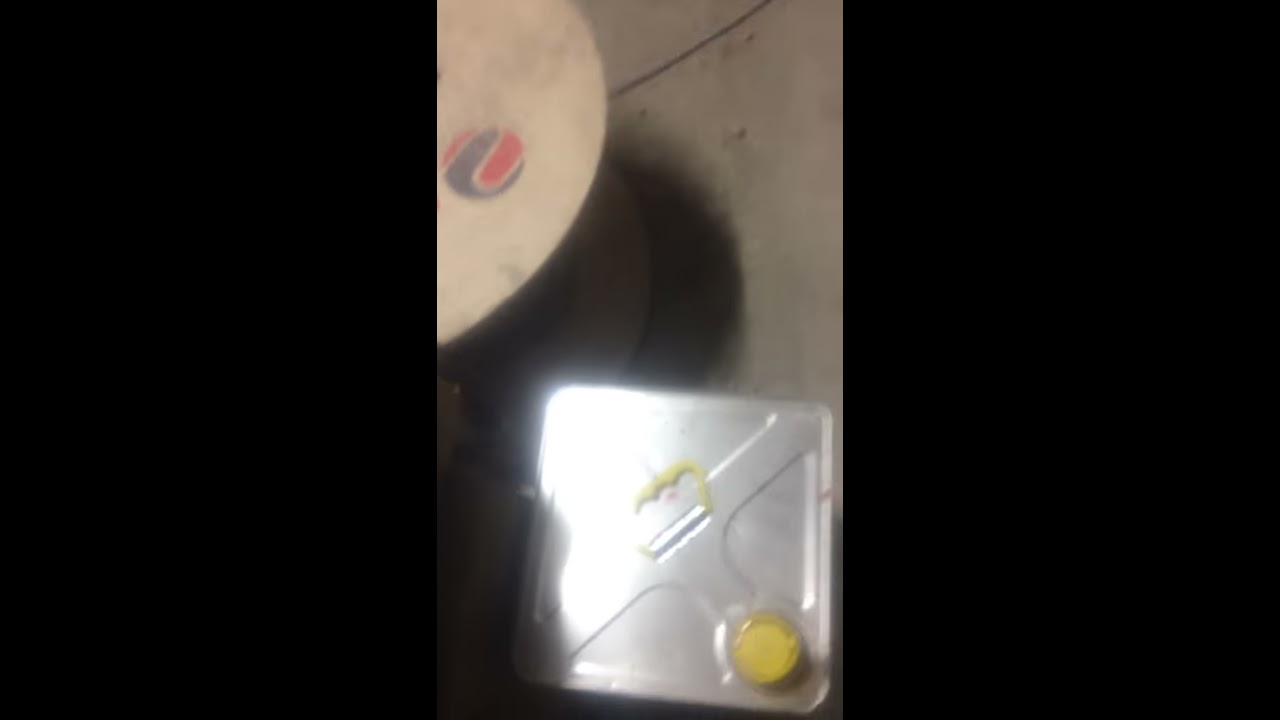The image, framed in thirds with the left and right sides letterboxed in black, showcases a top-down view onto two distinct objects resting on a wooden floor. Dominating the lower middle section, we see the metallic top of a square tin container, potentially an oil or gas can, featuring a small yellow twist-off cap centrally located and a larger yellow handle. This container is bathed in glare from a light source, enhancing its metallic sheen. To the upper portion of the image, there's a partial view of a large wooden spool, with its right side prominently displayed. The spool bears a red and blue circular logo intertwined on its top surface, and casts a pronounced shadow onto the floor beneath it. The overall composition is detailed, capturing the textural contrast between the smooth metal of the tin and the rustic wood of the spool.